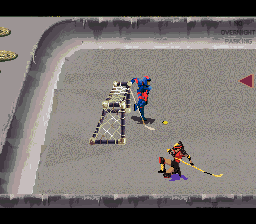This image is a highly detailed screenshot from a retro 90s-style video game, showcasing a unique hockey arena set in a rectangular pit with rounded edges. The pit, bordered by gray cement, appears to be embedded in a street and flanked by the partial view of two bicycles with yellow wheels. The arena itself has a distinct gray, concrete-like surface with black spots, encapsulated by a thin, dark frame. In the center, a dynamic hockey game unfolds with a visible yellow puck. On one side, a goal framed in blue with white netting is seen, featuring a goalie donned in a blue and red outfit with orange markings, wielding a brown hockey stick. Opposite the goalie, a player in red, yellow, and black attire is sprawled on the ground, possibly injured, with a mysterious blue color emanating from her leg area and her stick lying nearby. This small, square image captures the nostalgic pixelated charm and intense action of a bygone gaming era.